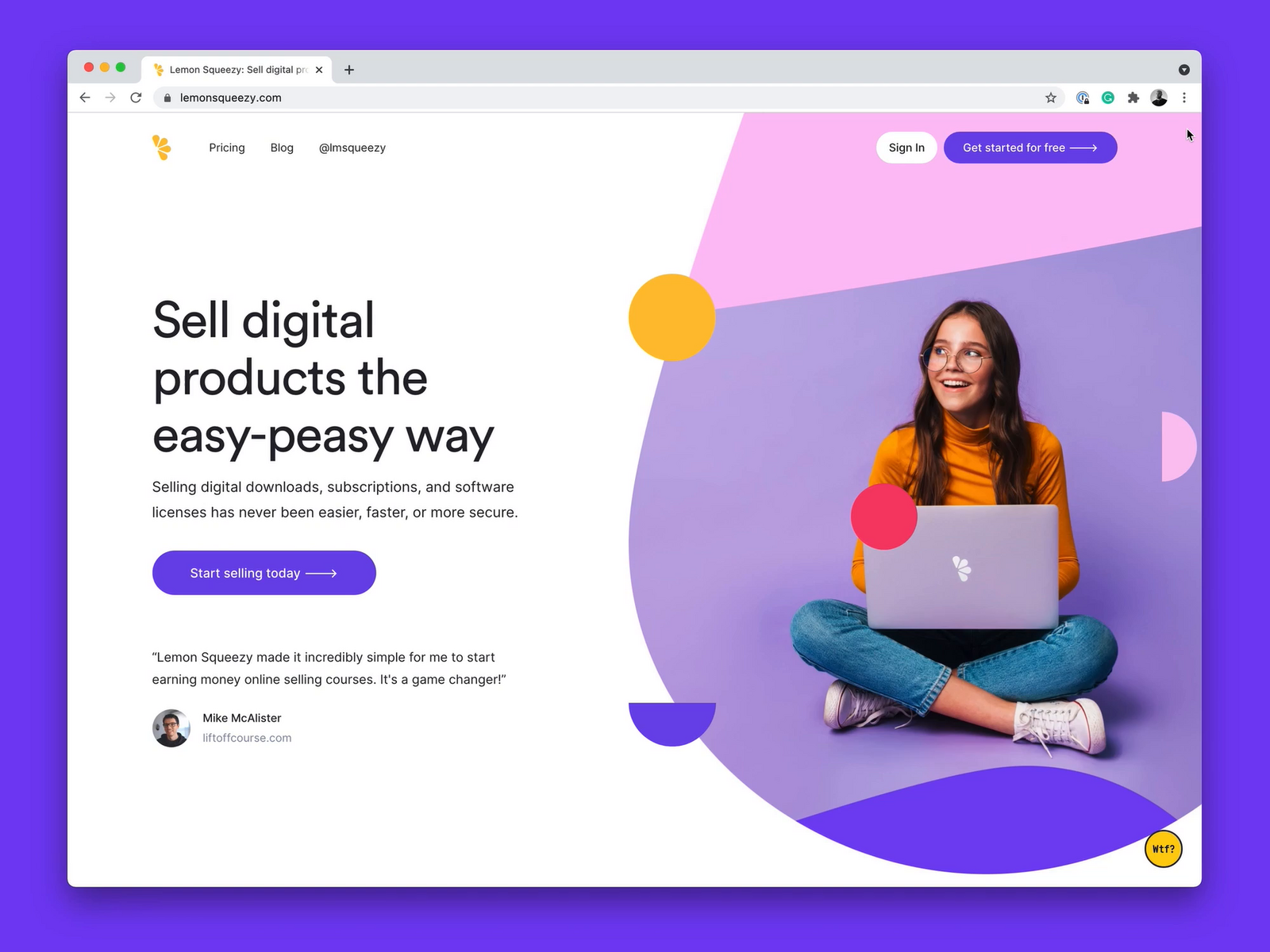The image features a computer screen displaying a web page from a Mac computer, identifiable by the red, yellow, and green control buttons in the upper left corner. The screen, framed by a medium purple border, shows a single open browser tab. The website being visited is "lemonsqueezy.com."

At the top of the webpage, a logo comprised of four yellow pin-like icons, reminiscent of Google Maps markers arranged in a half-circle with the tapered end pointing outward, is depicted. To the right of the logo are three horizontal menu options in black text: "Pricing," "Blog," and "About Lemon Squeezy." The webpage has a white background.

The main section of the webpage contains large black text in the center that reads, "Sell digital products the easy-peasy way." Beneath this headline, slightly smaller black text announces, "Selling digital downloads, subscriptions, and software licenses has never been easier, faster, or more secure."

Following this information is a prominent purple button with white text stating "Start selling today" accompanied by a right-facing arrow. 

Further down, a testimonial is quoted in black text: "Lemon Squeezy made it incredibly simple for me to start earning money online selling courses. It's a game changer." This quote is accompanied by a picture of the testimonial giver, identified as Mike McAllister.